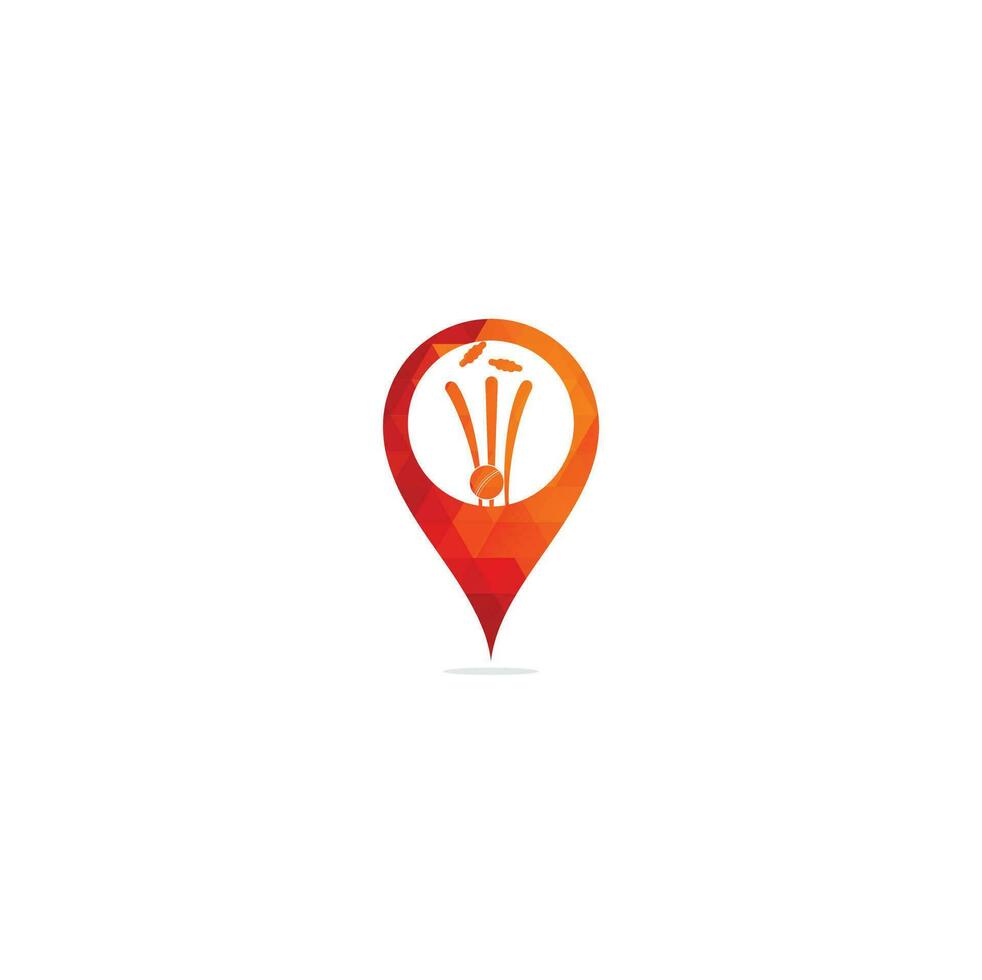The image features an upside-down teardrop shape reminiscent of a GPS pin drop, tapering to a sharp point at the bottom. Its color transitions from a dark red at the base, through various shades of red and orange, to a burnt orange and yellow toward the top. On the left side, the shape is predominantly red, while the right side is more yellow. Central to the teardrop is a large white circle, inside which an orange circle anchors three orange lines radiating upward in different directions. Above these lines are two small, oblong, cloud-like orange shapes: one oriented horizontally and the other diagonally. The teardrop casts a gray shadow beneath it, all set against a white background, devoid of other elements.